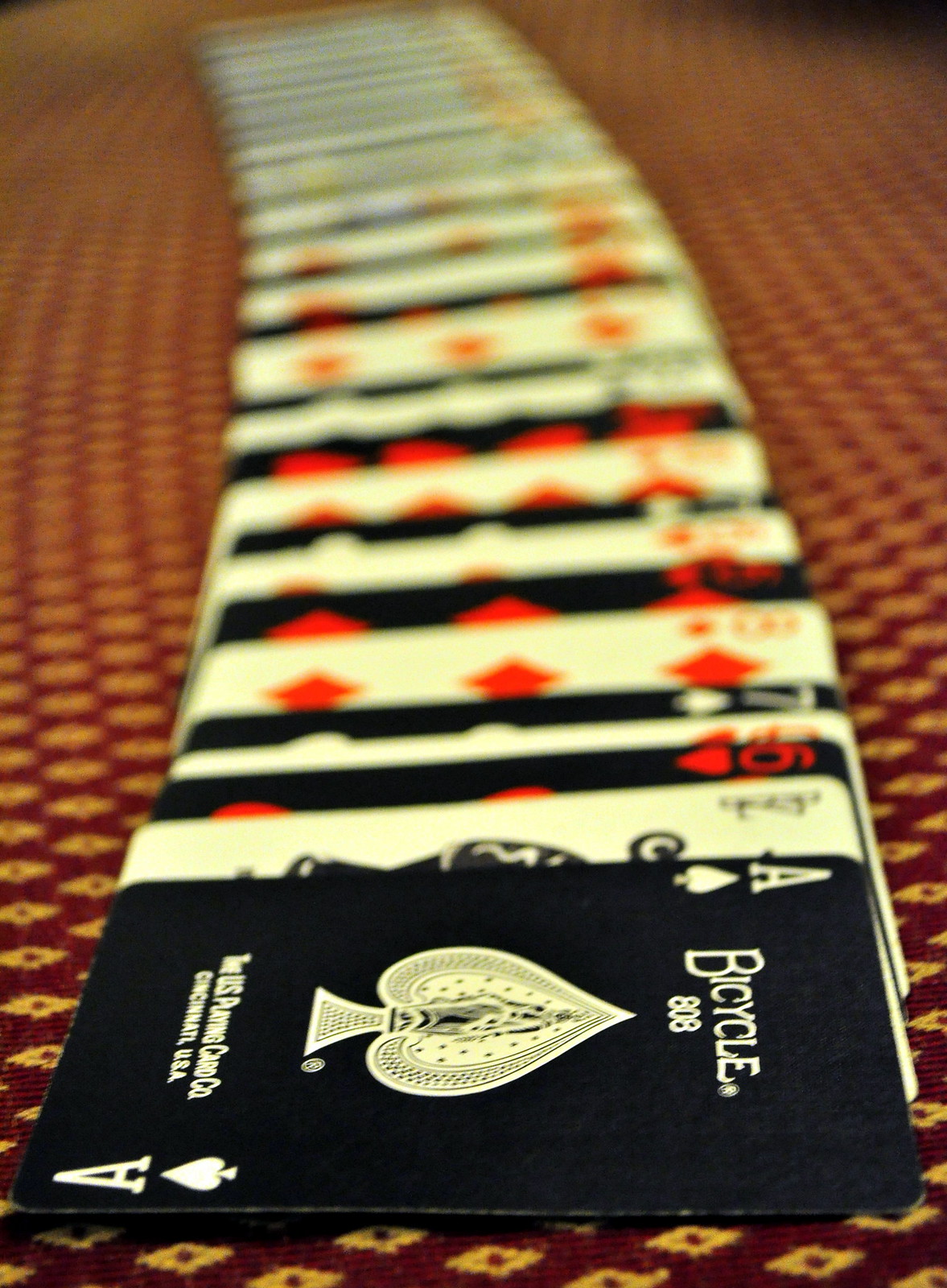This color photograph captures a meticulously arranged deck of playing cards displayed on a table with a richly textured maroon tablecloth adorned with an intricate pattern of gold diamonds. The eye is immediately drawn to the ace of spades situated at the bottom center of the image. This card, part of the renowned Bicycle brand, features a black backdrop with a distinctive white "A" and spade symbol, underlined by the iconic "Bicycle" logo at the top. While the cards extend across the frame from bottom to top, most of the photograph is enveloped in a gentle blur, keeping the focus primarily on the ace of spades. The adjacent cards, including the five of hearts to the immediate right and the three of diamonds slightly further up, are partially discernible amidst the soft-focus ambiance, contributing to the image's elegant and somewhat enigmatic visual narrative.